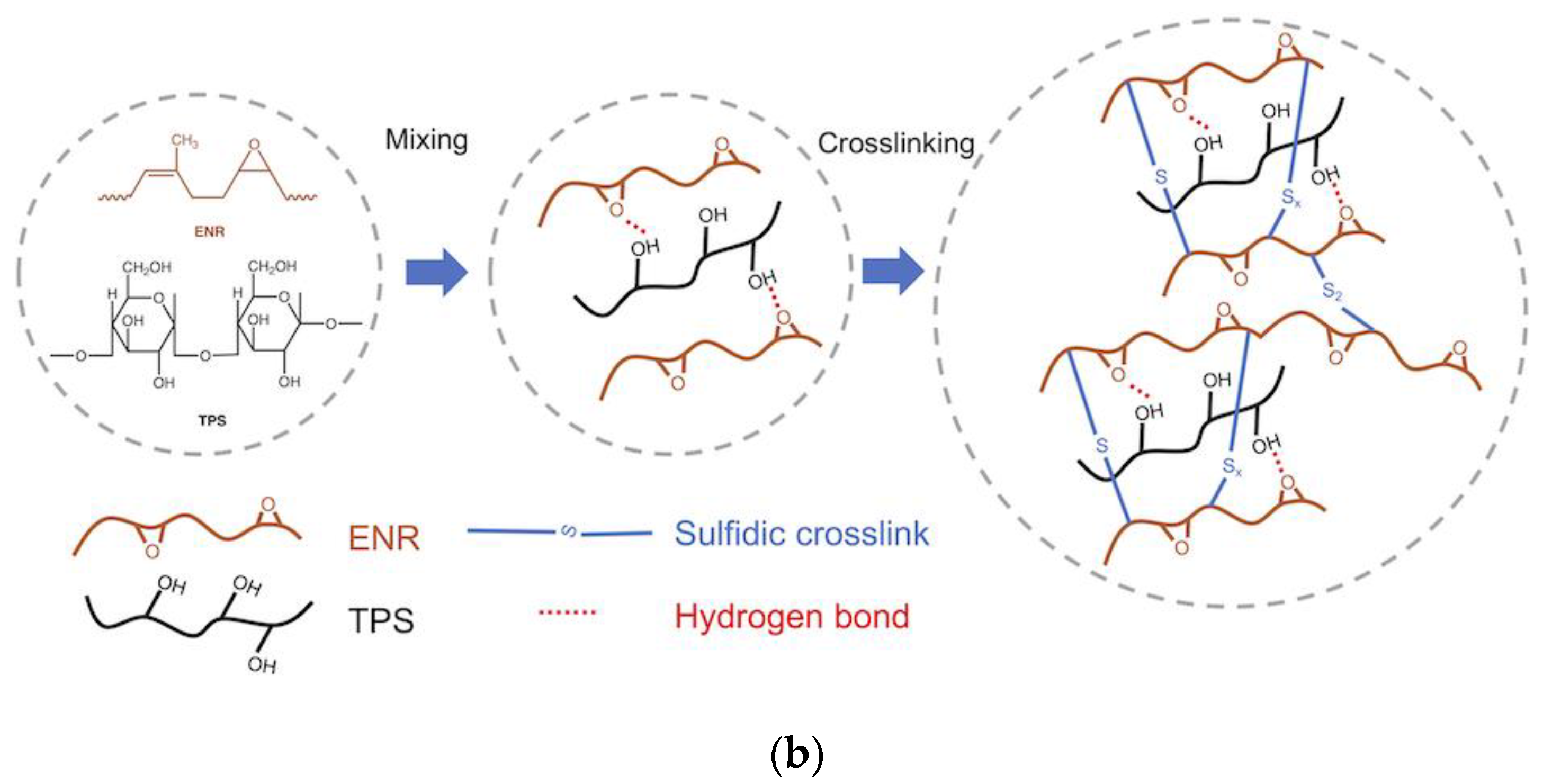This is a detailed scientific diagram illustrating stages of a chemical reaction through a series of three interconnected circles with dotted gray outlines. The first circle on the left depicts various chemical shapes, including symbols representing oxygen and chloride. Accompanying it is a blue arrow labeled "mixing," which points to the middle circle. The middle circle, also dotted, contains additional chemical diagrams with wavy lines in brown and black, representing different chemical bonds. Another blue arrow labeled "cross-linking" leads to the largest circle on the right. This final circle presents an intricate illustration of the fully linked chemical structures.

Beneath the circles, there is an index with a detailed explanation of symbols. This legend includes ENR (depicted with brown lines), TPS (depicted with black lines), and descriptions of sulfidic cross-link and hydrogen bond interactions. The letter "B" in parentheses is also noted at the bottom of the index, which further clarifies the diagram components. Overall, the diagram visually explains the mixing and cross-linking processes in a chemical reaction, emphasizing the shapes, bonds, and stages involved.